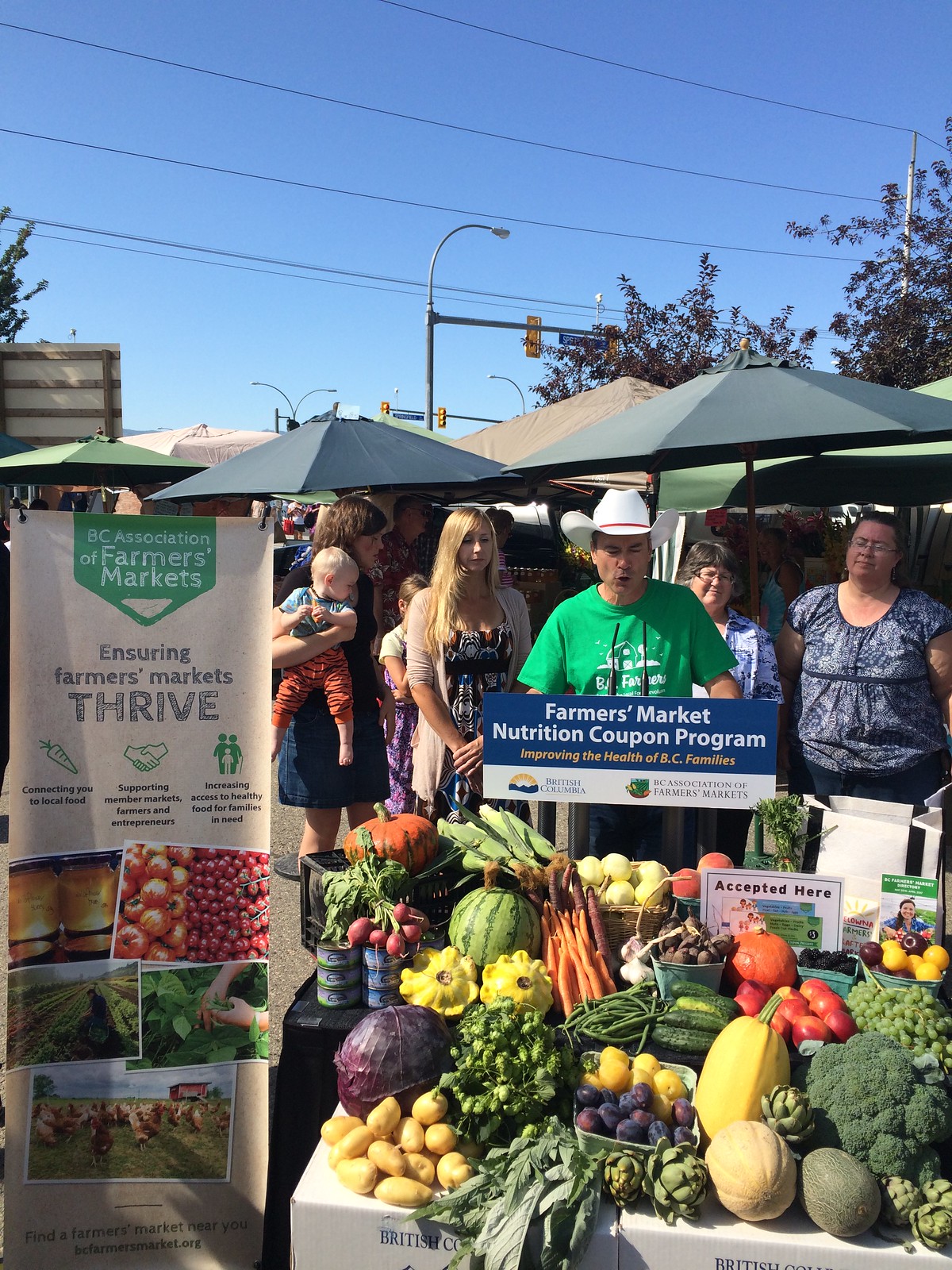This vibrant and colorful outdoor photo captures the lively atmosphere of a farmer's market on a sunny day. Beneath a clear blue sky, tables laden with a variety of fresh produce burst with colors: oranges, yellows, greens, purples, and reds. Fruits and vegetables such as potatoes, cabbage, squash, melons, broccoli, oranges, apples, tomatoes, carrots, watermelons, beets, radishes, lemons, and grapes fill the scene. In the bottom right of the image, produce is arranged meticulously on a table. Adjacent to this table, an advertisement reads "Farmer's Market Nutrition Coupon Program, Improving the Health of BC Families," alongside another sign that says "BC Association of Farmers Markets, Ensuring Farmers Markets Thrive."

At the center, to the right, a man wearing a green T-shirt with lettering and a white cowboy hat is holding a sign featuring the same text as the advertisement. He is surrounded by people: to his left, two women in blue blouses, and to his right, a woman holding a child and another woman. The people are under colorful umbrellas—blue, tan, and green—that provide shade for the stands below.

Above the market scene, the blue sky continues, dotted with trees and crisscrossed by telephone lines. In the distance, a yellow stoplight blends with the greenery of the trees, enhancing the vibrant community feel of the market scene. The entire image embodies the charm and vitality of a bustling farmer's market on a beautiful day.